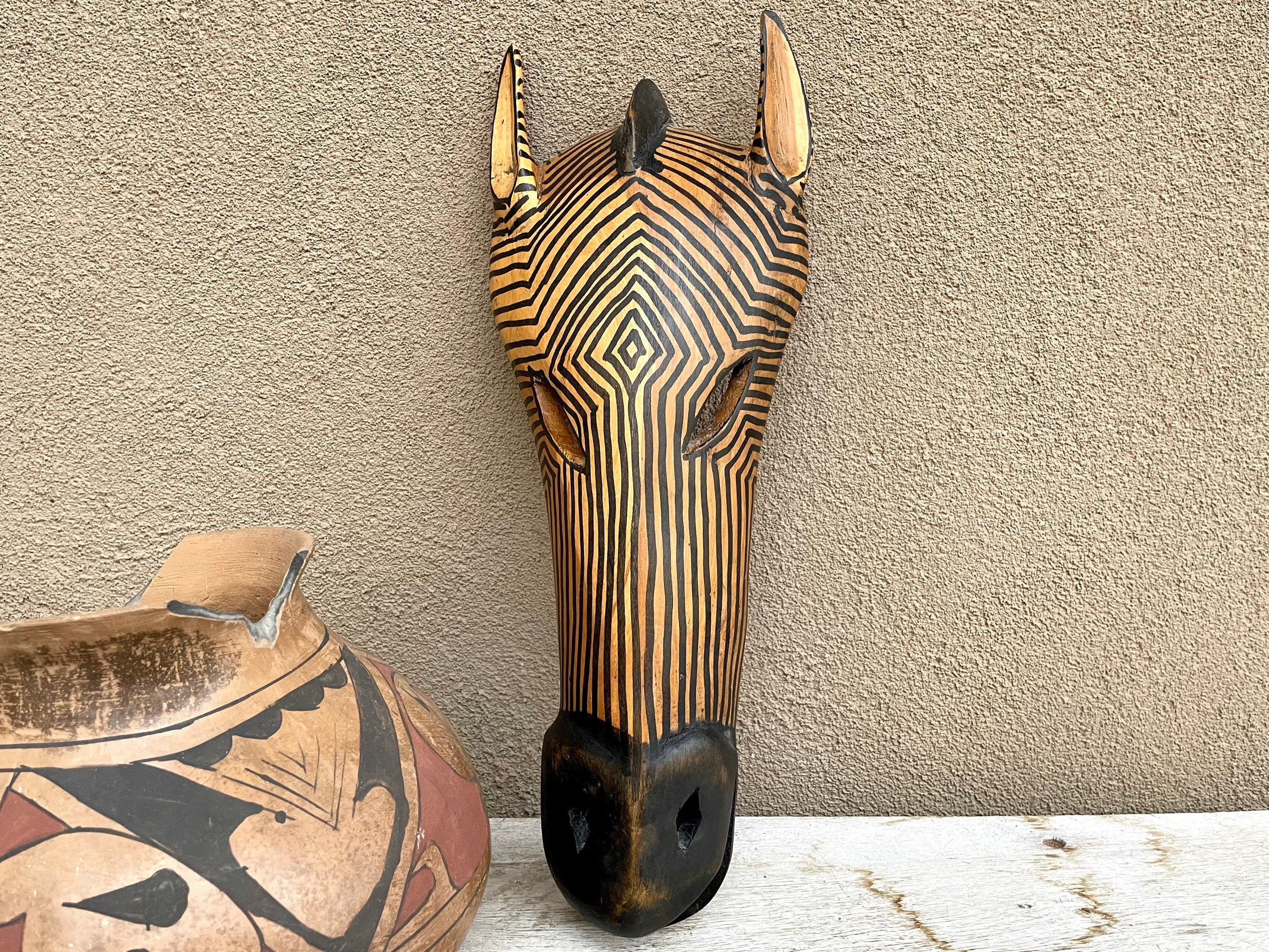This color photograph captures two remarkable pieces of art displayed on a white surface with a beige wall in the background. On the lower left, there is an old vase or bowl, light brown in color with intricate black and red designs that suggest a tribal or ethnic origin. The bowl is chipped at the top but features a rounded lip, indicating that it might have been used to store and pour water. 

Next to the bowl is a beautifully carved animal face, possibly representing a zebra due to its long snout, large nostrils, slanted eyes, and small pointed ears on the top. The sculpture appears to be made of wood or bone and is painted with black and gold stripes, resting on the white surface while leaning against the beige wall. The eyes are notably hollowed out, adding a striking detail to the piece. Together, these objects create a visually compelling scene, likely captured in a museum or an exhibit space, highlighting both the artistic craftsmanship and cultural significance of these artifacts.